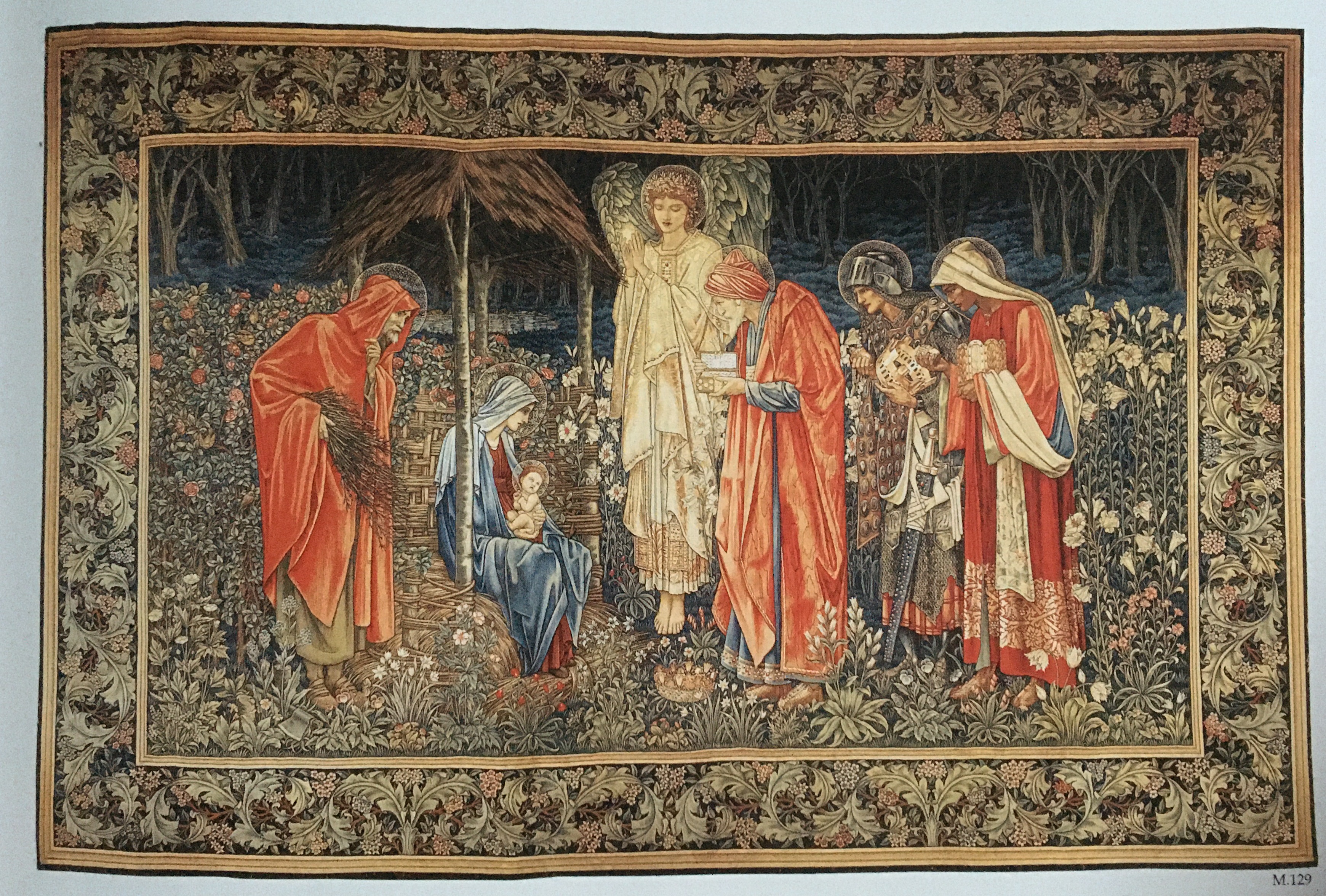This detailed photograph captures a richly depicted religious tapestry with a muted floral and green leaf background. The tapestry centers on a Nativity scene, showcasing Mary holding the baby Jesus, while Joseph, appearing to hold straw or wood, stands protectively beside them. Surrounding the Holy Family are the three wise men, adorned in vivid red, white, and darker robes, bearing gifts for the Christ child. Dominating the center, an angel clad in white with wings spreads a radiant light over the scene. The figures are arranged under a stable, giving a sense of sacredness and shelter. The tapestry is framed by a floral border, enriching the overall composition with intricate gold and brown hues. The setting evokes the dark, humble atmosphere of Bethlehem, contrasted by the ethereal illumination from the baby Jesus and the angel, effectively portraying the profound reverence of this biblical moment.